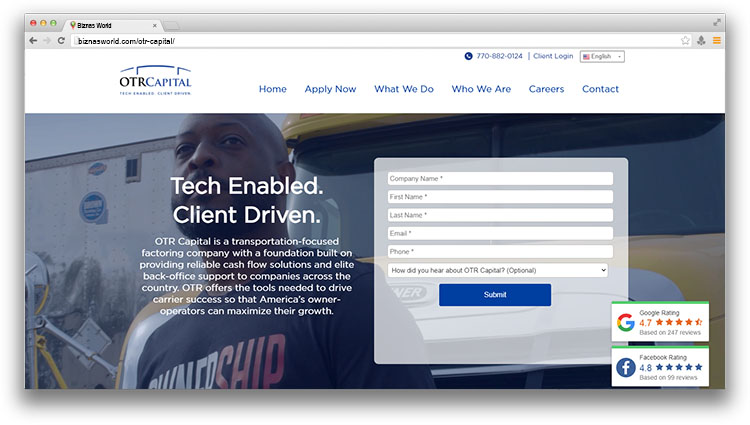This screenshot captures a web page from an internet browser, specifically the URL "businessworld.com/OTR-capital/". The image features the OTR Capital website, showcasing a clean and professional layout.

At the top, there's a wide white header displaying the OTR Capital logo, consisting of "OTR" in black and blue letters, followed by "Capital" in black. Above the text is a half-circle bridge icon. Within the header, there's a menu with links in blue text: "Home," "Apply Now," "What We Do," "Who We Are," "Careers," and "Contact." Additionally, there is a client login option and a language selection toggle.

The main content area features a background image of an African American man wearing a shirt that appears to say "Ownership." Overlaying the image are bold white letters reading "Tech Enabled. Client Driven." Below this slogan is a paragraph detailing OTR Capital's services.

On the right side of the page, there's a form for visitors to fill out, requesting their company name, first name, last name, email, and phone number. There is also a dropdown menu for selecting how they heard about the page, culminating in a "Submit" button set over a grey box positioned atop the background image.

In the bottom right corner, the web page displays a Google rating and a Facebook rating, providing quick access to user reviews.